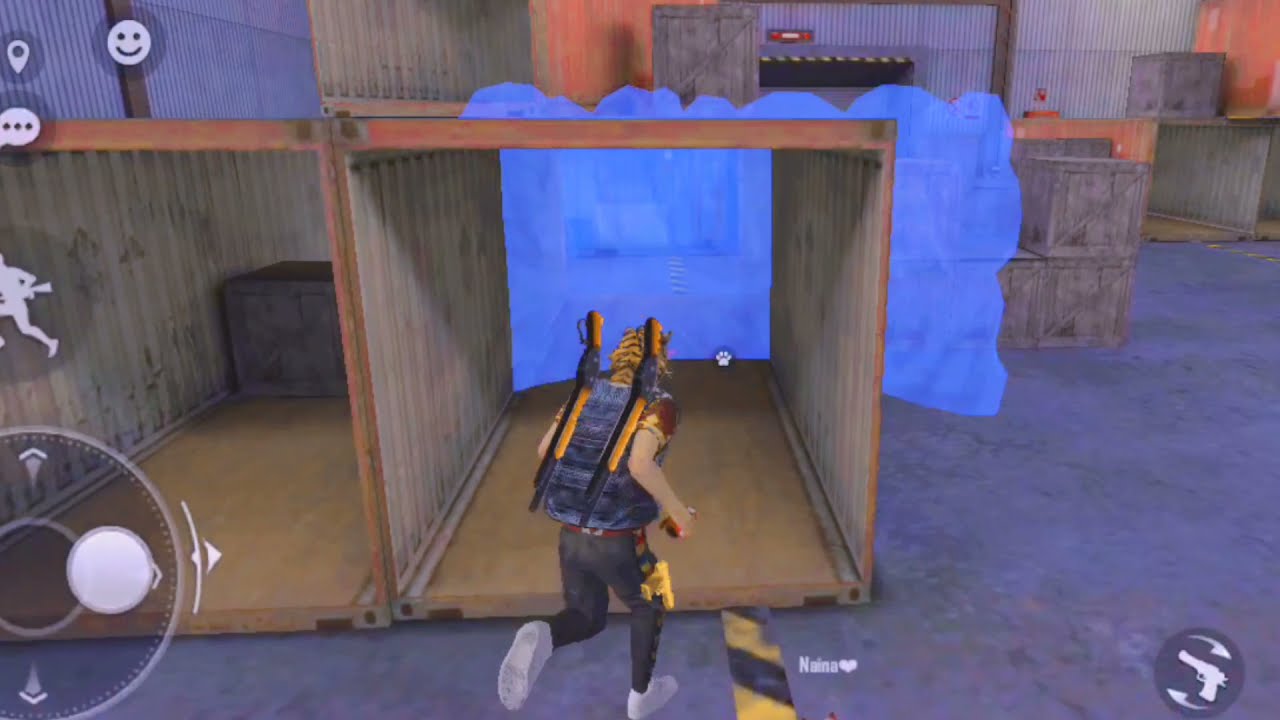This screenshot from a video game appears to be taken from a mobile device, displaying various controls on the screen. In the bottom left, there's a semi-transparent directional pad with a white joystick in the center, along with buttons featuring a speech bubble, a location marker, and a happy face. On the bottom right, there's a semi-transparent circle with a white outline of a gun inside.

The scene features an animated figure running away from the camera into a large, open shipping container with a brown interior. The character is dressed in black pants, a black vest, white sneakers, and has two shotguns strapped to their back. Interestingly, the character's hood has a pattern resembling tiger stripes, adding a unique detail to their appearance. 

The surroundings depict an industrial warehouse or loading dock environment, with more shipping containers stacked together in the background. These containers are variously wooden, gray, and orange. Additionally, a large, semi-transparent blue cloud-like shape spans the interior and part of the exterior of the central shipping container. The ground is gray, and in the distance, there's a metallic wall that resembles a garage door. Inside another similar shipping container to the left, a brown box is visible.